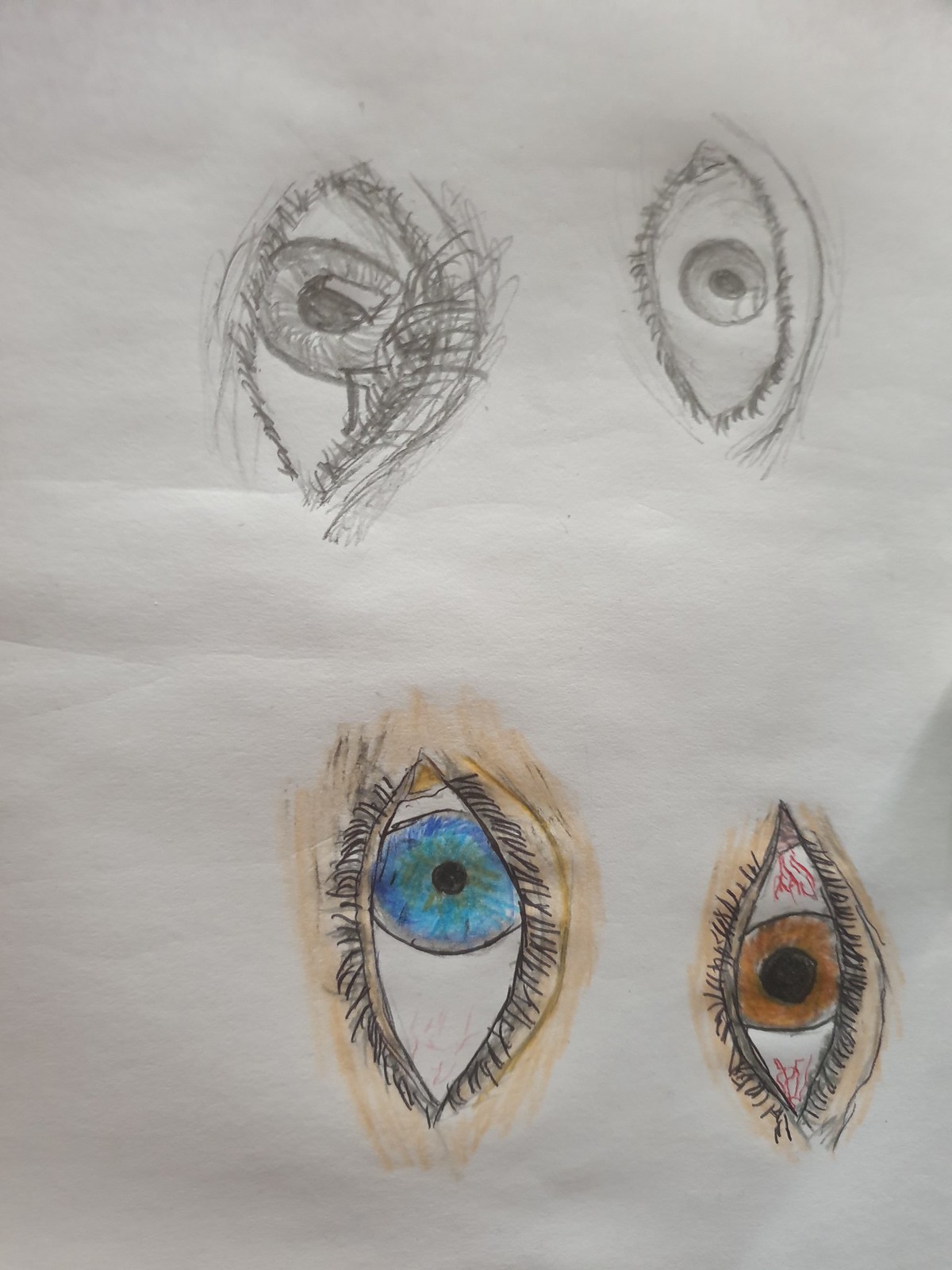This image features four distinct eyeball illustrations arranged vertically. The two eyeballs at the top are pencil sketches, devoid of any color. The left one, with an enlarged iris and elongated eyelashes, appears larger than the adjacent right one. Both top illustrations are intricately drawn, highlighting careful pencil work. 

The bottom two eyeballs are colored; the left one is a vivid blue eye, while the right one is a deep brown. Although the blue eye is slightly larger, both eyes have similarly short eyelashes, measuring approximately a quarter-inch in length. Both eyeballs are distinctly white, with the blue eye displaying a subtle thin red vein at the bottom. In contrast, the brown eye is marked by prominent, bright red veins that branch out on all sides—top, bottom, left, and right—enhancing the vividness of the illustration.